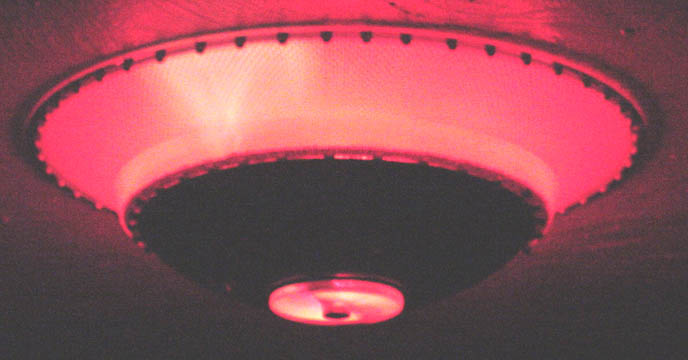This image is a horizontally oriented color photograph featuring a unique, ceiling-mounted light fixture with a dome shape. The larger, circular base of the light is secured to the ceiling with a series of black screws around its white or light glass rim, which occupies the outer third of the fixture. From this base, a black, convex dome protrudes downward, narrowing slightly. In the center of this black dome is a small, clear glass circle, held in place by a single black screw, allowing light to pass through it. The entire scene is cast in a dark red hue, giving the image an unusual, otherworldly appearance. The light primarily emits through the larger area attached to the ceiling, but also through the clear glass center of the dome. The background remains dark red, enhancing the dramatic effect of the red light being emitted. The photograph represents realism and captures the intricate details of this distinctive light fixture against a simple ceiling backdrop.